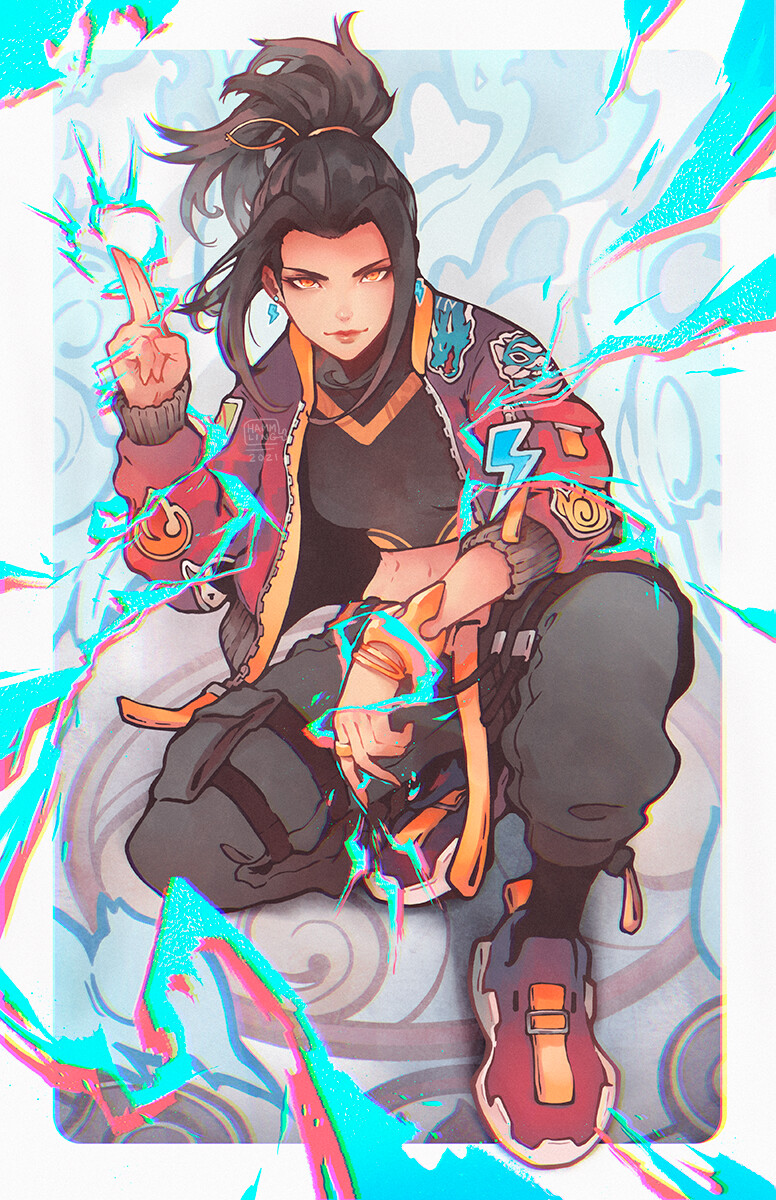The vertical rectangular image features a full-body depiction of an animated female character positioned centrally. She has black hair with brown tips, styled into a ponytail secured with a brown hair tie, and face-framing strands falling by the sides. The character's attire includes a black shirt with an orange V-neck, topped by a bomber jacket with dark maroon or brown shoulders transitioning to a red body, and brown cuffs. The jacket is adorned with various patches; notable ones include a turquoise animal near her neck on her left arm, another turquoise animal, a red pouch with an orange buckle on her right sleeve, a lightning bolt, and a penguin on her left elbow.

She strikes a dynamic pose: her left hand holds her first two fingers up and together while her thumb secures the other fingers, her elbow bent. Her right arm hangs down between her legs as she crouches. Her right knee is bent, revealing dark gray or black pants with black straps, and she wears black socks. Her shoes are red, transitioning to a black-purple shade near the toes, with a yellow tongue and vertical black lines resembling eyes. Her left leg is tucked lower to the ground, making its sneaker barely visible, accompanied by a gray or black pouch fastened with darker straps. The background is a visually engaging swirl of turquoise, white, and red hues.